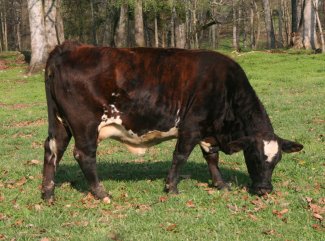In this small horizontal daylight image, a cow is standing in an open, grassy field, leaning forward to graze on the ground where there are leaves scattered, suggesting it might be fall. The cow is predominantly black with notable features including a big white spot on its forehead and a white underbelly. Additionally, there are specks of lighter brown, almost orangey, along its sides and a bit of white on its legs. The cow’s posture indicates that it was walking and paused to eat, with its two front legs and two back legs separated. Its tail is hanging straight down. The background features a lot of trees, forming a wooded area that frames the field. Overall, the scene conveys a sense of calmness as the cow peacefully grazes.